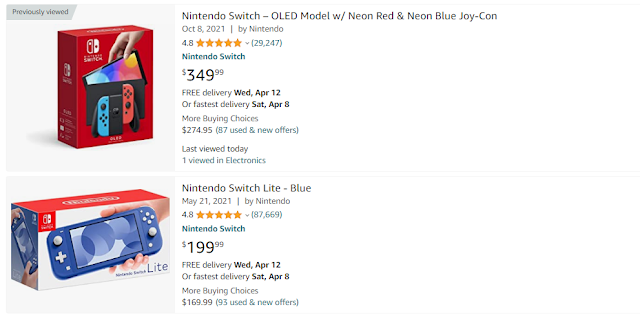The image features two Nintendo Switch consoles available for purchase. The first item, labeled as "previously viewed" in the upper corner, showcases a Nintendo Switch OLED Model. The console comes in a vibrant red box, alongside a detachable Joy-Con controller set in neon red and neon blue colors. The central image depicts a hand extracting a colorful cartridge from a case, highlighting shades of blue, purple, red, and yellow. This Nintendo Switch OLED Model is rated 4.8 stars and is priced at $349. Free delivery is available by Wednesday, April 12th, with an option for faster delivery by Saturday, April 8th.

The second item displayed is a Nintendo Switch Lite, a handheld gaming console that is designed to be played exclusively in handheld mode. The packaging box prominently exhibits the device in a blue hue, with the same image repeated on the side and bottom of the box. Released on May 21, 2021, by Nintendo, this Nintendo Switch Lite also boasts a rating of 4.8 stars and is priced at $199.99. Like the first item, free delivery is available by Wednesday, April 12th, or faster delivery by Saturday, April 8th.